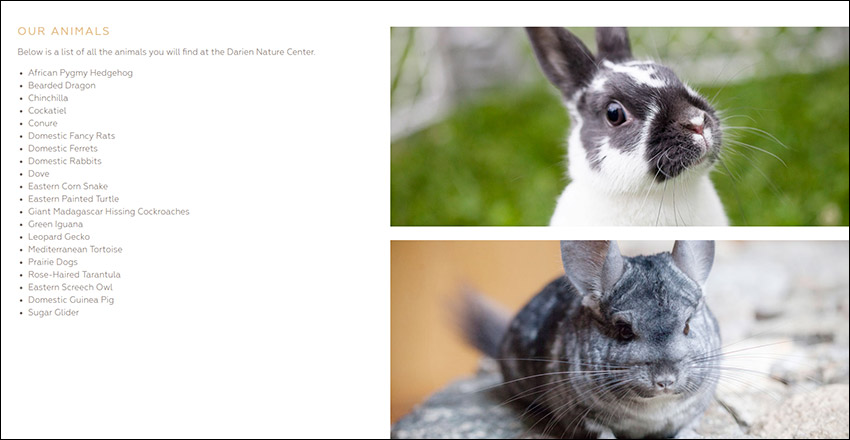The image appears to be a screenshot from a computer display, showcasing a detailed informational graphic. The display is divided into two primary sections. On the left side, against a white background, there is an extensive list of text, formatted into bullet points. The caption at the top reads: "Below is a list of all the animals you will find at the Darien Nature Center." The list includes:

- African Pygmy Hedgehog
- Bearded Dragon
- Chinchilla
- Cockatiel
- Conure
- Domestic Fancy Rats
- Domestic Ferrets
- Domestic Rabbits
- Dove
- Eastern Corn Snake
- Eastern Painted Turtle
- Giant Madagascar Hissing Cockroaches
- Green Iguana
- Leopard Gecko
- Mediterranean Tortoise
- Prairie Dogs
- Rose-Haired Tarantula
- Eastern Screech Owl
- Domestic Guinea Pig
- Sugar Glider

On the right side of the graphic, there are two images. The top image features a black and white rabbit with distinctive dark grayish-black ears, black markings around its eyes and nose, and white fur on its cheeks, chest, and the back of its head. This rabbit is set against a background of blurry grass and a chain-link fence. The bottom image depicts a gray chinchilla sitting on a rock. The chinchilla has lighter and darker gray fur, with the darker hue more prominent between its eyes. Although its tail can be seen in the background, it appears blurry.